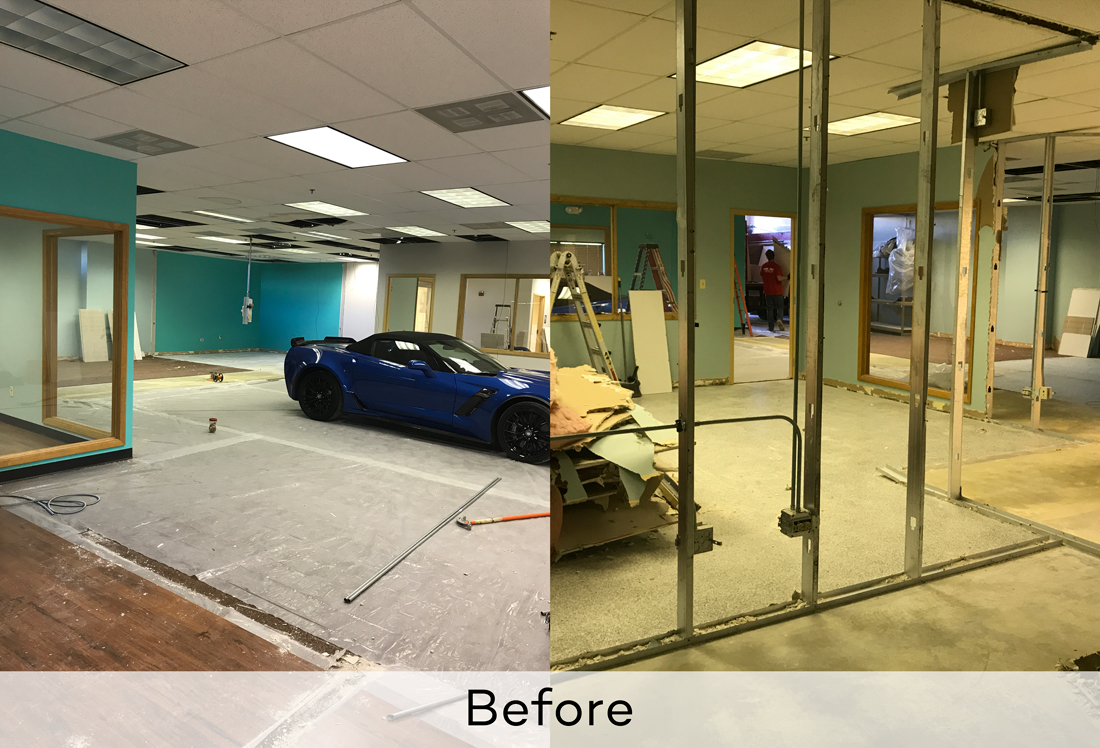This composite image showcases two distinct views of a large, cavernous space undergoing significant remodeling. On the left, we see an area with a wooden floor shielded by a gray tarp, where a blue sports car is conspicuously parked mid-right. The ceiling features typical office elements like white panels interspersed with fluorescent lights. The partially exposed teal and white walls have missing window frames and doors. 

The right side of the image provides a different angle, capturing a more yellow-tinted view of the ongoing construction. The space is stripped to the metal framing, with drywall removed, revealing the light green interior walls. The floor in this section is a brownish-beige, littered with construction tools such as wooden ladders and materials, alongside cluttered refuse on pallets to the left. A person in a red shirt and blue jeans can be spotted in the background. Unaltered areas are demarcated by a gray border along the bottom, featuring centered black lettering. This dual-view effectively illustrates the stark contrast of the space both before and during its extensive renovation process.